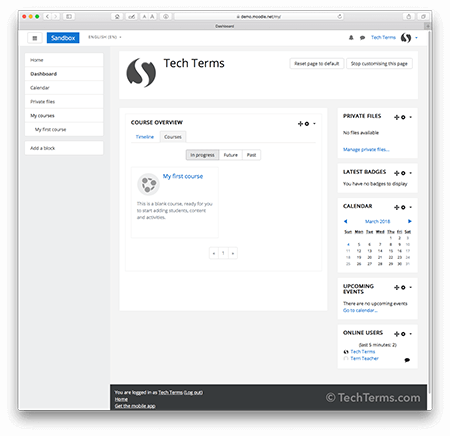A detailed screenshot of a computer display showcases a section of the TechTerms.com website, specifically a course overview titled "Tech Terms." The interface features a right-hand sidebar displaying various elements including "Latest Badges" and a "Calendar." The text, though small, includes some entries in blue writing, adding a hint of interactivity or hyperlinks, typical of modern educational platforms. The branding "TechTerms.com" is visibly prominent, reinforcing the identity of the website.